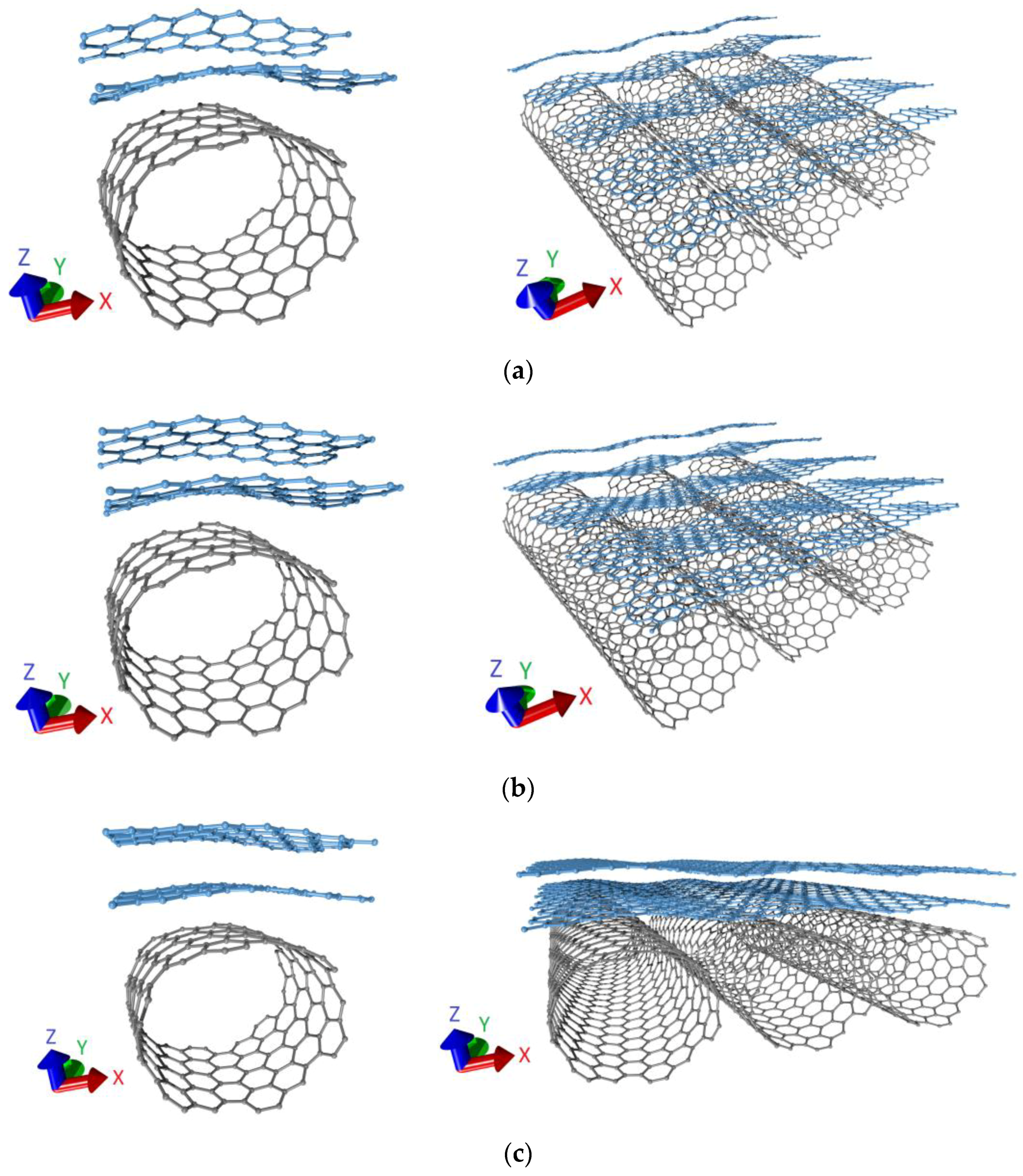The image is a detailed scientific diagram showcasing the structure of carbon nanotubes. It consists of six sub-images arranged in two columns and three rows, labeled A, B, and C from top to bottom. The left column illustrates smaller, circular pieces of dark gray, hexagonally arranged carbon nanotubes, each with a set of axes markers at the bottom left (X in red, Y in green, and Z in blue). Arrows labeled X, Y, Z point toward these tubular structures. The right column presents a more zoomed-out view, displaying three elongated carbon nanotube segments in each sub-image, overlaid with flattish hexagonal blue sheets. These blue layers in the images appear to be distinct and are floating above the nanotubes, emphasizing the multi-layered composition. The diagram, set against a white background, provides various perspectives and layers of the carbon nanotubes, likely for an in-depth product explanation or scientific analysis.